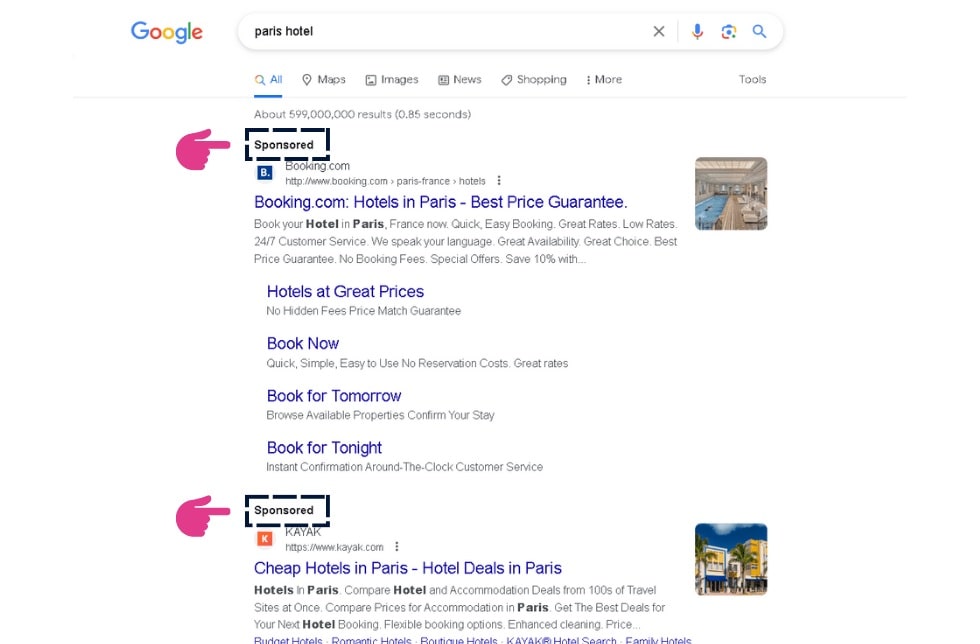This screenshot captures a Google search results page for "Paris hotels." The familiar multi-colored Google logo is prominently displayed in the upper left-hand corner. Just below, the search bar reads "Paris Hotel." Beneath the search bar are several filter options: All, Maps, Images, News, Shopping, More, and Tools.

Highlighted in the search results are sponsored entries, marked by a purple icon shaped like a pointing finger. The first sponsored entry is outlined by a black dashed rectangle and features Booking.com. This entry promotes "Hotels in Paris Best Price Guarantee" and includes booking options for "Hotels at Great Prices" with enticing calls to action: "Book Now," "Book for Tomorrow," and "Book for Tonight." To the right of this entry is a small, indiscernible square photo.

Below the Booking.com link is another sponsored entry, similarly marked with a pointing finger icon. This entry features Kayak and advertises "Cheap Hotels in Paris" along with "Hotel Deals in Paris." Adjacent to this entry, on the far right, is a square photograph showcasing a yellow building set against a blue sky.

Collectively, these elements illustrate a visually organized and user-navigable interface designed to aid users in discovering the best hotel deals in Paris.